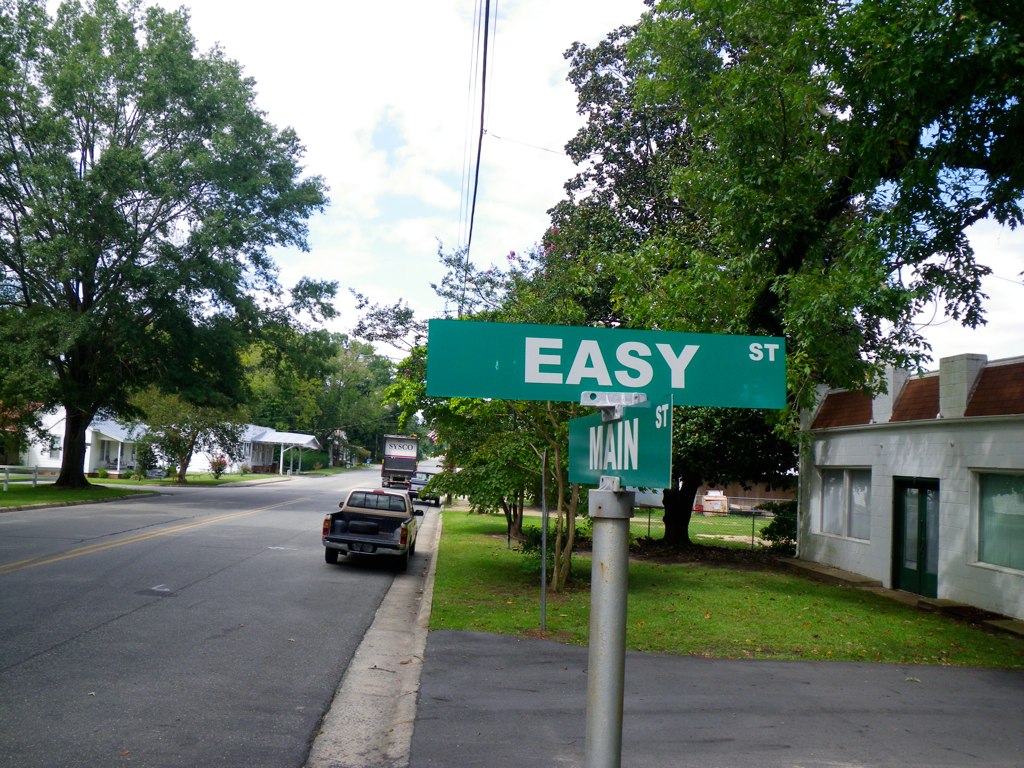The photograph captures a suburban street corner under a clear blue sky. A road runs from the bottom left towards the middle of the image, lined with trees on both sides. In the upper left, there are two white houses at the edge of the road. To the right of the road, a silver pickup truck with its tailgate down is parked, and further in the distance, what appears to be a moving truck or a U-Haul is visible, parked near a tree line. A driveway comes in from the right, past a light-colored concrete gutter, and intersects with the road. A small house with a white front, a brown roof, and a black door with two big windows flanks the bottom right corner.

Dominating the center of the image is a silver pole with a pair of green street signs. The top sign, facing the viewer, reads "Easy St" in white letters. Perpendicular to it is another green sign indicating "Main St." The corner is characterized by lush greenery, with a grassy area and a large tree near a white building with a red rooftop and double windows. Just behind the driveway, on the right, is another tree and a yard. The distant background features additional parked vehicles, including a black and white delivery truck, and a blue and silver truck, emphasizing the suburban setting.